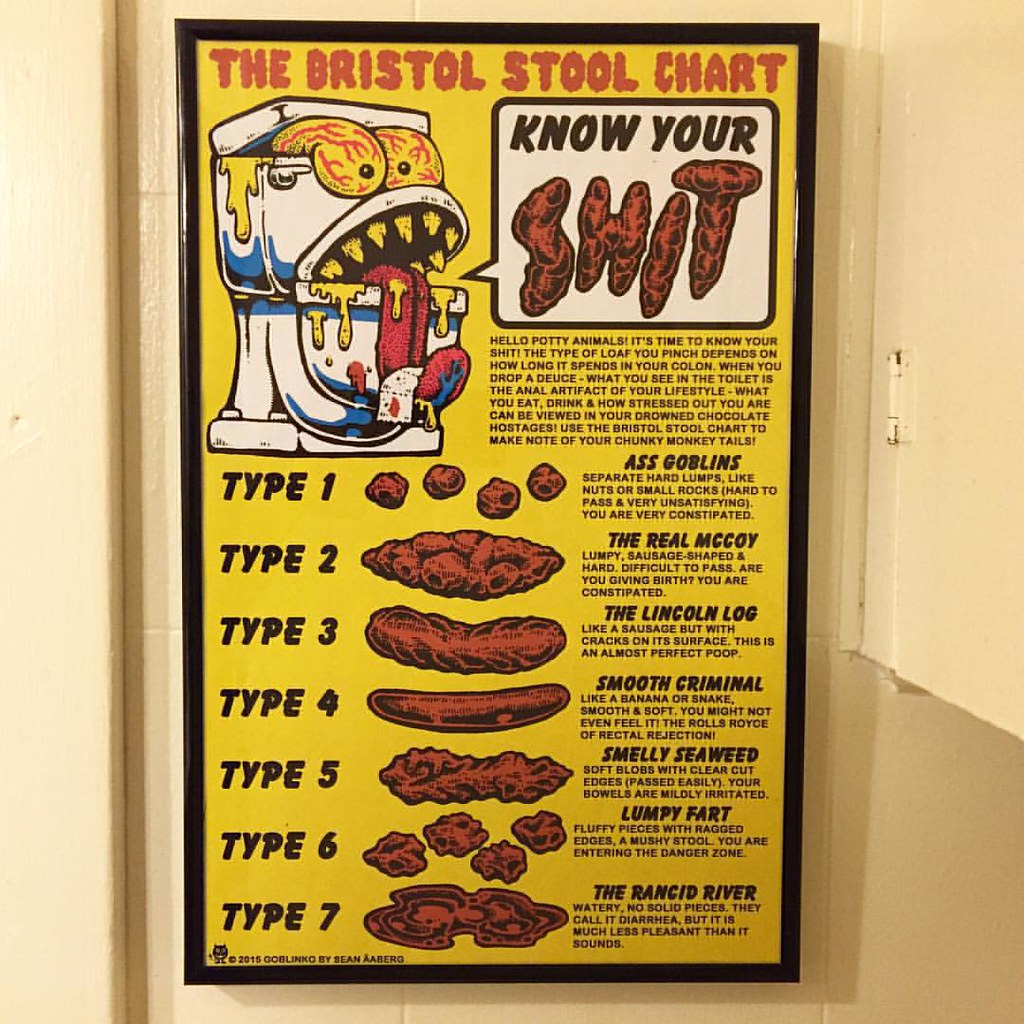This image is a color photograph in portrait orientation, capturing a bathroom interior with light tan walls. Dominating the center is a vertical poster framed in black. The poster's background transitions from yellow at the top to red, with bold black text. The headline reads "The Bristol Stool Chart," introducing an educational and humorous take on different types of bowel movements. In the top left corner of the poster, a cartoonish white toilet is illustrated as a monster, complete with bulging yellow eyes with red veins, a wide-open lid as a mouth, dripping red teeth, and a long red tongue adorned with a piece of toilet paper. To the right of this whimsical toilet is a black-outlined speech bubble with the text "Know your" in black and "Shit" in brown, crafted from illustrations of feces. Below the speech bubble, a paragraph offers a playful yet informative narrative about bowel health, emphasizing the importance of understanding one’s stool. The lower section of the poster features a detailed chart of seven types of poop, each accompanied by descriptive titles and illustrations running vertically from top to bottom. Types range from "Type 1: Ass Goblins" depicting small, hard lumps, to "Type 7: Rancid River," illustrating watery diarrhea. Each type includes humorous and vivid descriptions, providing insight into potential digestive conditions. In the lower left corner of the poster, there is a small circular devil figure with the text "© 2015 Goblinko by Sean Aaaberg," tying in the artistic credit.